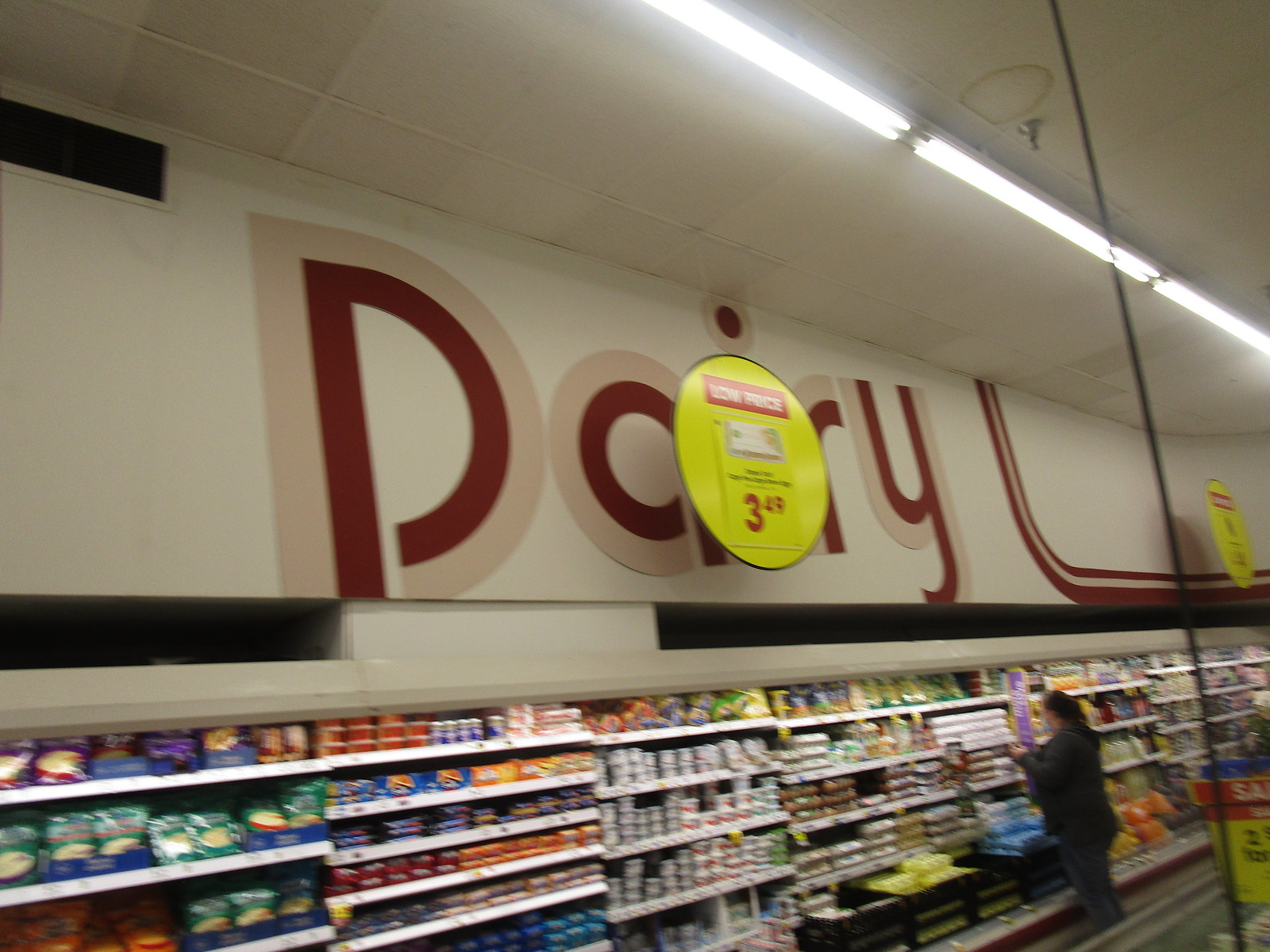In this slightly blurred image, the dairy section of a grocery store is prominently featured under the bright glow of fluorescent ceiling lights. The centerpiece is a large, eye-catching sign that reads "Dairy" in contrasting burgundy and pale pink letters, hanging above the well-stocked and brightly illuminated shelves of merchandise. A woman, dressed in a long-sleeved dark shirt and matching dark pants, stands facing the egg section, her dark hair flowing down her back. Suspended in the foreground, a circular yellow sign draws attention with a red rectangle, showcasing the white-lettered phrase "Low Price," and prominently displays the price of $3.49 in bold red numerals below some additional writing. The image captures a moment of everyday life within the bustling, organized environment of a grocery store’s dairy aisle.